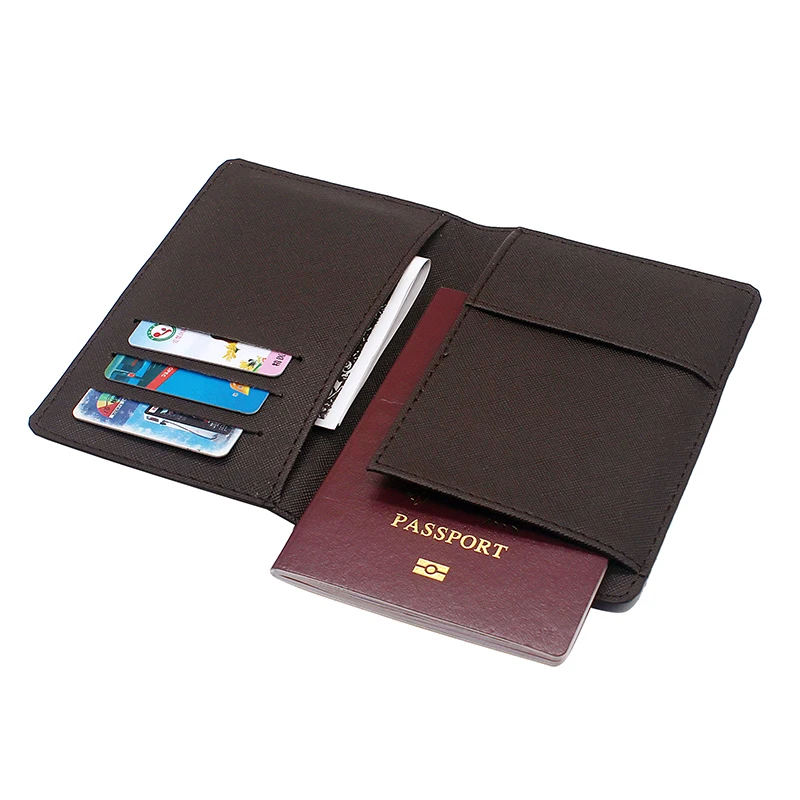This is a detailed image of an opened bifold wallet, prominently featuring its rich brown, textured, leather-like material. Positioned diagonally on a white background, the left side showcases three card slots, each containing a credit card. Below these slots, there's a pocket partially revealing folded paper currency. The right side highlights a passport compartment, with a burgundy passport cover, embossed with gold lettering, sliding out from the bottom. Additionally, there are other shallow compartments for storing various small items, making it a functional and organized accessory.